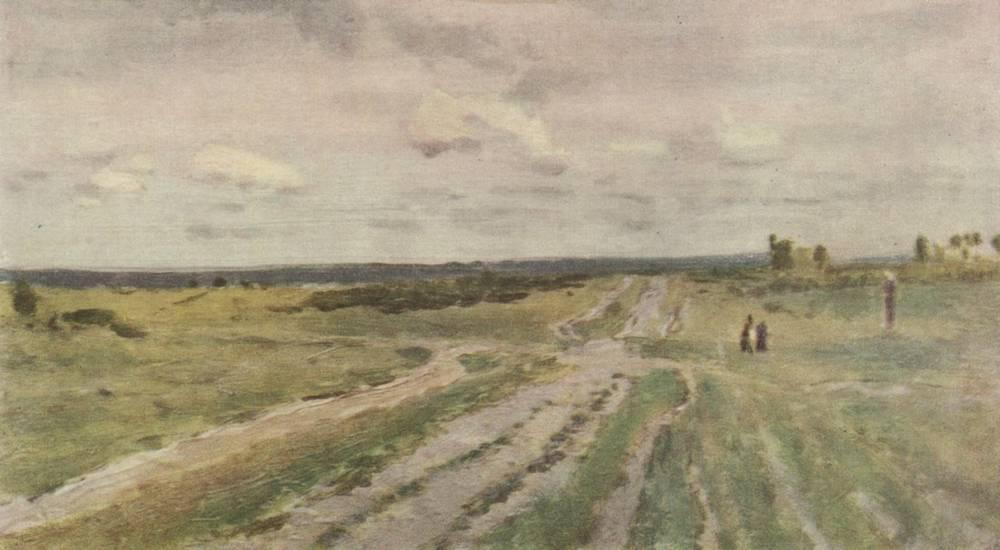This painting, titled *The Vladimir's Road* by Isaac Levitan, created in 1892, is a color oil painting in a realistic landscape style. The artwork portrays a somber and dimly colored landscape, emphasizing the natural and rugged elements of the scene. The central focus is a field with a dirt road cutting through the center, bordered by patches of green shrubs, grass, and bushes amidst uneven stretches of bare earth. This road converges toward the horizon just right of the center, deepening the illusion of depth.

In the foreground, patches of green and dirt interweave, appearing almost unhealthy and sparse. To the right, there are three human figures—two squatting and one standing—amidst the greenery and trees. The background transitions into a rocky area, followed by a distant tree line and what might be a body of water or more indistinct landscape features, all set against a gray sky filled with billowy clouds, conveying a rather dreary or overcast day. The overall atmosphere painted by Levitan is one of realism infused with the subtle melancholy of a gray, cloud-covered sky.